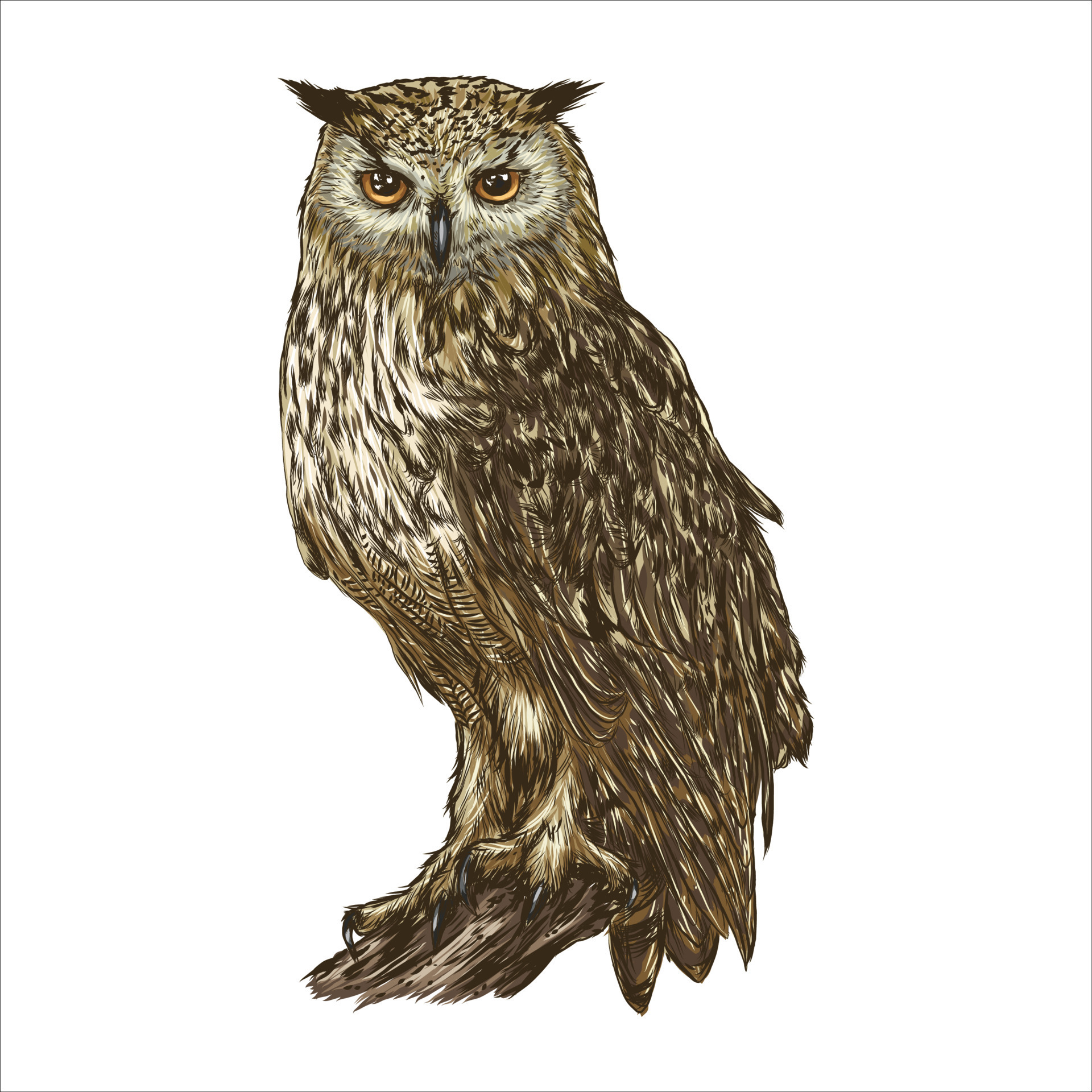This is an illustration of a majestic horned owl perched on a tree branch, set against a completely white background with no additional details or watermarks. The owl, depicted with remarkable realism, features tufts of feathers above its eyes tipped in black, adding to its striking appearance. Its feathers are a mix of darker and lighter brown, with hints of white on its chest, and they appear somewhat messy and interwoven, particularly on the back. The owl's vivid orange irises and large black pupils, which reflect light in a unique pattern, lend a captivating and lifelike quality to its gaze. The thin, black beak and sharp talons gripping the branch are meticulously detailed, enhancing the realistic feel of this pen and ink-style drawing. Overall, the illustration showcases the owl in a powerful and engaging manner, making it appear almost alive to the viewer.